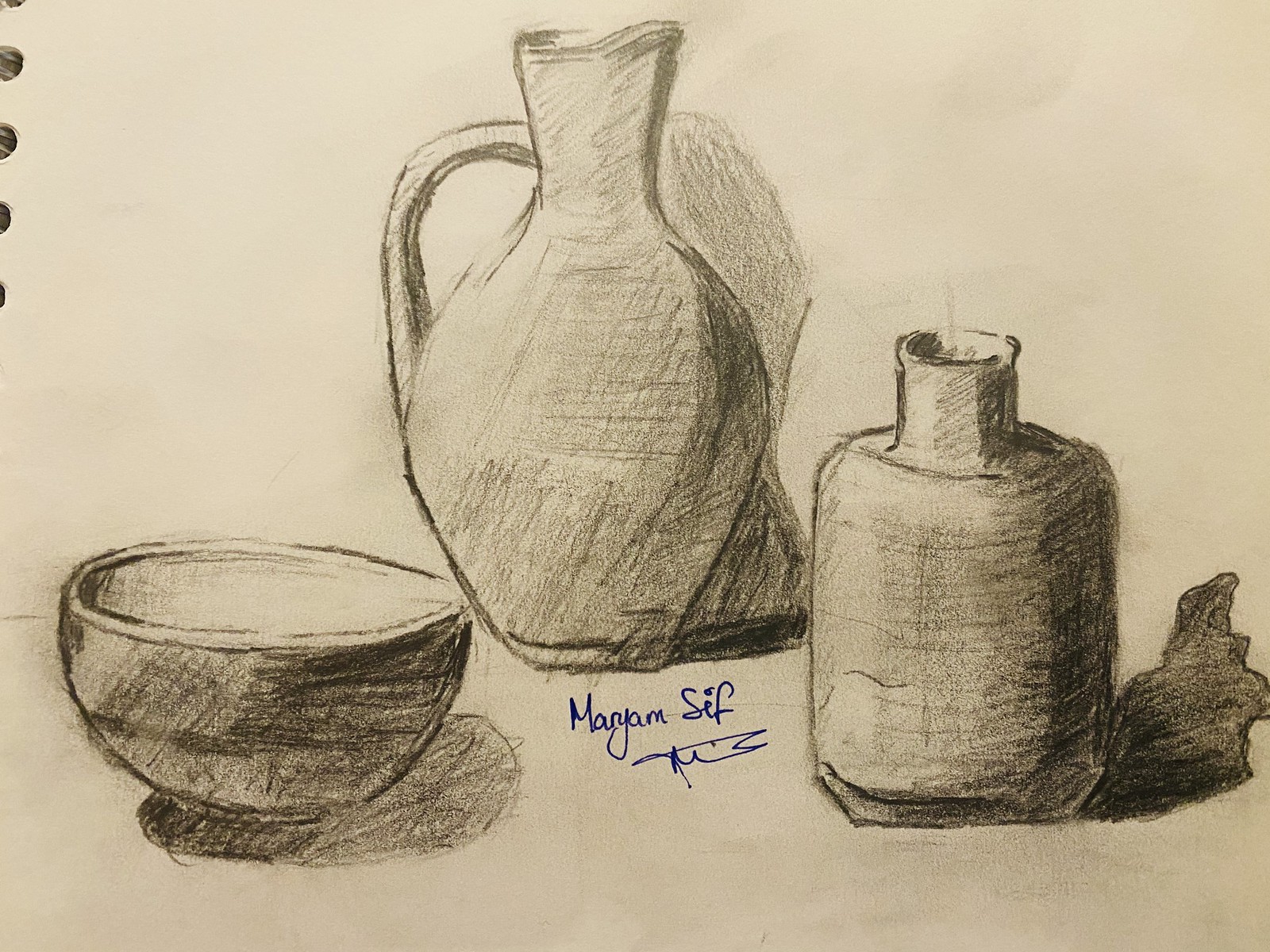The image depicts a pencil sketch on plain, notebook-style paper, which has holes along its edge similar to those found in printer paper. The artwork, housed in the notebook, features three distinct containers. The first container is a small bowl with simple, clean lines. The second container resembles a pitcher, identifiable by its visible handle. The third container looks like a vase but is rather small and includes a protruding tube at its top center. The sketch is signed in blue ink with the name "Marion Sif Maryam," followed by the initials "M.S." Each container casts a distinct shadow, enhancing the depth and realism of the drawing.